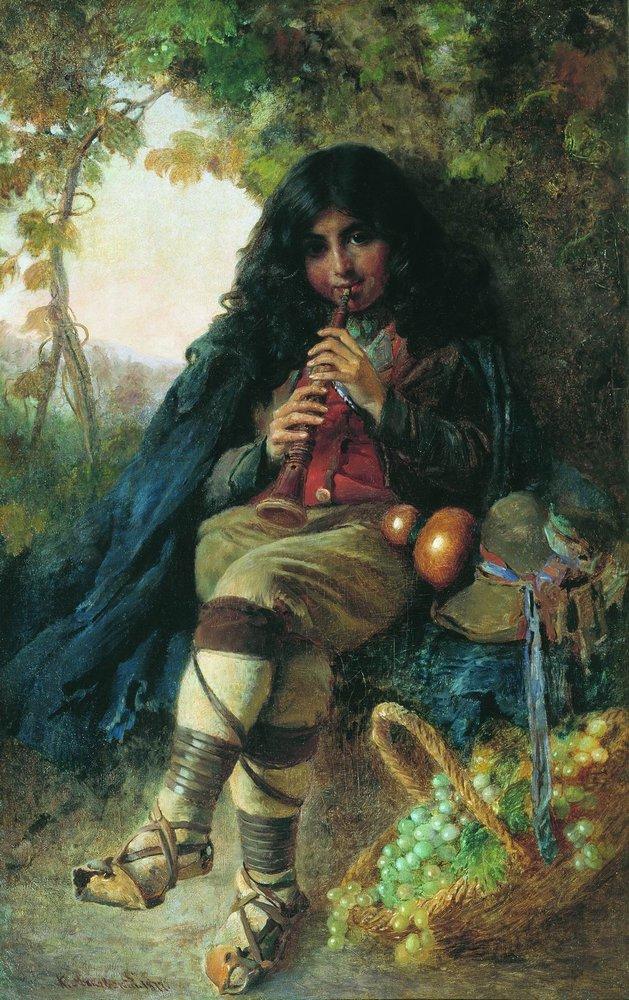In this detailed and evocative painting, a young girl with long black curly hair is depicted sitting in front of a tree. She is playing a wooden wind instrument, likely a clarinet, with a serious expression on her face. The girl wears a striking blue cape over a red button-up shirt, paired with beige pants that are adorned with brown leather ribbons at the knees. Her outfit is completed with brown shoes that lace up and wrap around her ankles like boots. In front of her rests a wicker basket overflowing with luscious green grapes, and to her side, a hat with a scarf tied around it adds a touch of elegance to the scene. The background is filled with greenery, vines, and a glimpse of the sky breaking through on the upper left side, enhancing the serene outdoor ambiance of this artwork. The painting exudes a timeless quality, suggesting a scene from a bygone era.